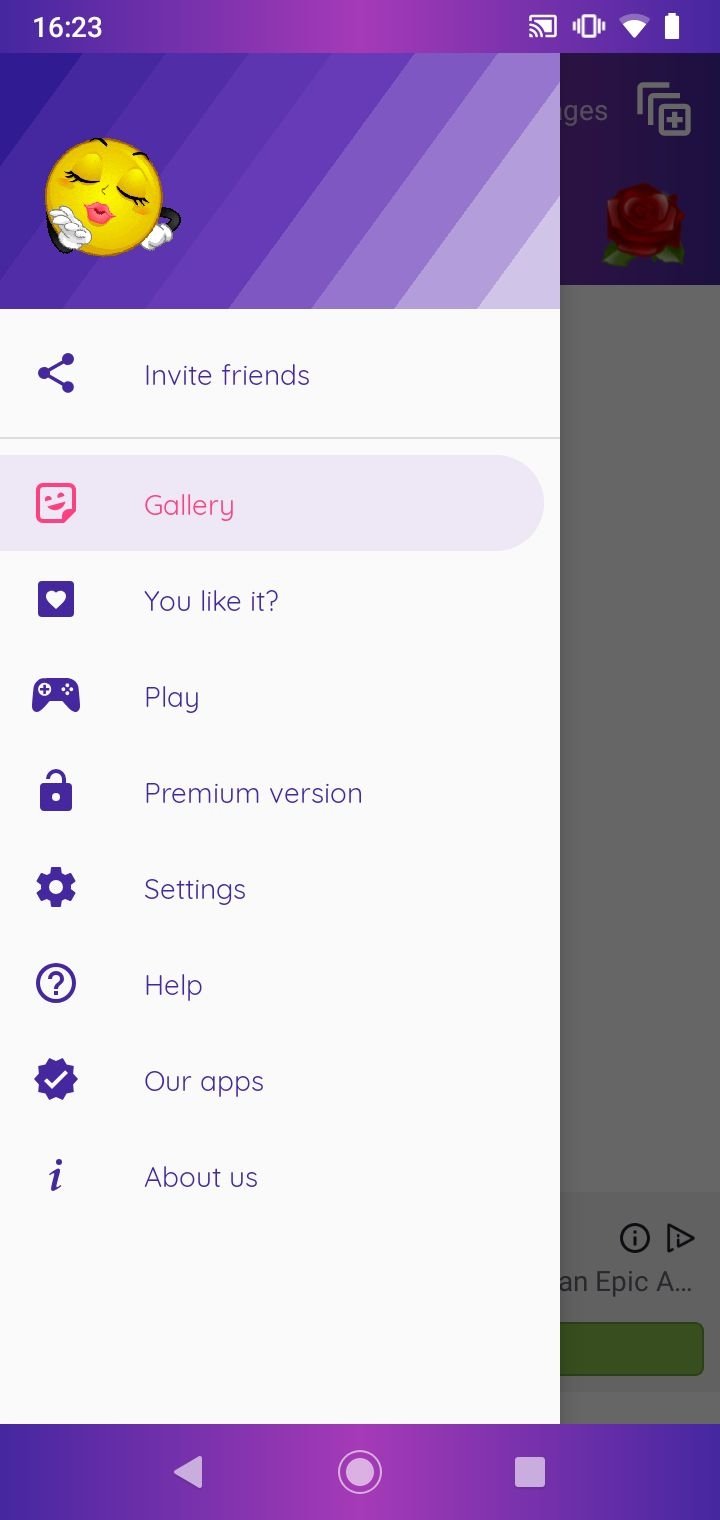This image is a screenshot of a mobile phone screen, captured at 16:23, as indicated by the white timestamp on the left side of the prominent purple bar at the top. On the right side of this bar, various icons are displayed in white: a screen share icon, a vibration status icon, a mobile signal strength icon, and a battery status icon.

Beneath the top bar is a visually striking purple rectangle adorned with diagonal stripes that transition from a darker to a lighter shade of purple from left to right. Positioned on the left side of this rectangle is a detailed yellow emoji featuring a pair of expressive eyes, well-defined eyebrows, and kissy lips, with small white hands blowing a kiss.

Immediately below this colorful rectangle is a sleek white vertical dropdown menu. The menu starts with a small share icon, followed by the text "Invite friends" in bold purple font. The next entry has an emoji icon adjacent to the word "Gallery" in gray font, highlighted by a light translucent purple bar, indicating it has been selected. 

Further down, the menu features a purple square icon with a white heart inside, accompanied by the text "You like it?" Next is an icon resembling a game controller, with the word "Play" displayed alongside it. Below this is an unlocked lock icon with the text "Premium version," suggesting advanced features are available. The final item on the menu is a gear icon labeled "Settings," signifying access to configuration options.